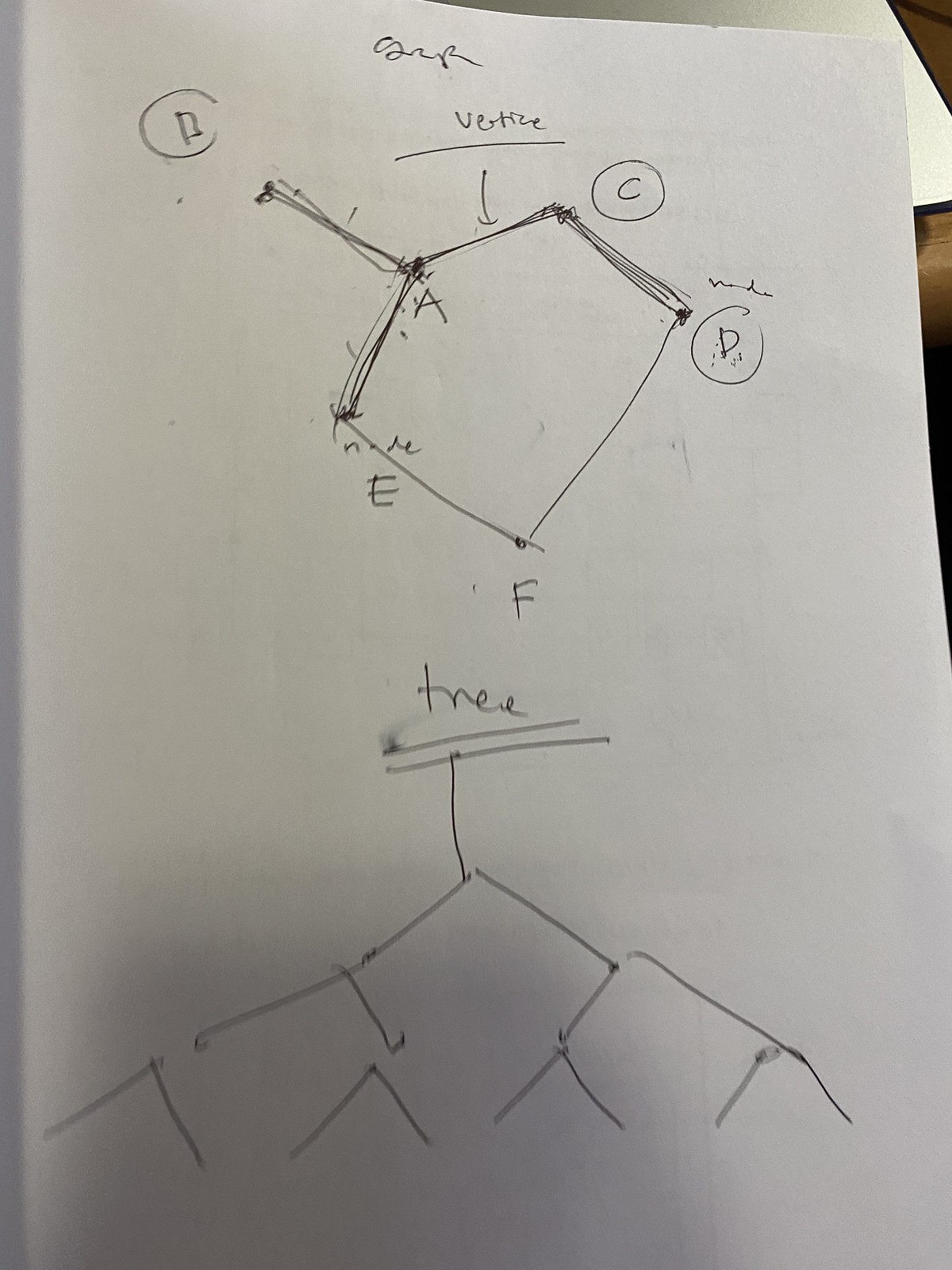The image depicts a detailed diagram drawn on a white sheet of paper, photographed at an angle. In the background, the top-right corner of the paper is visible, while the top-left corner is obscured. The paper appears to be placed on a desk, with part of another book or a white object partially visible in the frame.

On the paper, the diagram begins with a word at the top that is hard to decipher due to its cursive style, following which the word "vertis" is clearly written with a line underneath it. In the top-left corner of the diagram, there is a small circle containing the letter "B."

Below the "vertis" label, a polygonal object with five sides is depicted, ending in a point at the bottom. Each side of this object is marked with letters: A, E, F, D, and C. A line extends from the "A" point located at the top-left of the polygonal figure.

Further down the paper, the word "tree" is written, underlined with two lines. Below this, a vertical line extends downwards, branching out into multiple lines that resemble a root system. The branches of this root system spread outwards, with additional lines branching from them, creating an intricate root-like pattern.